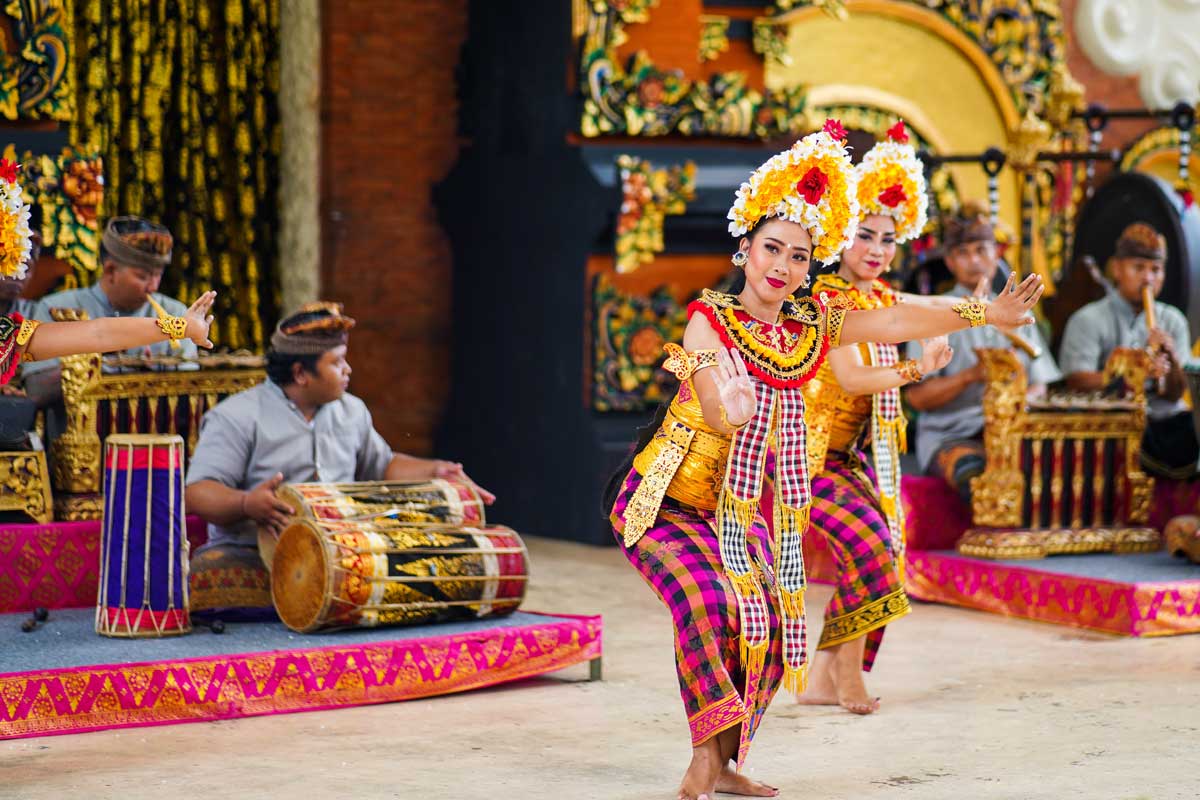In this vibrant outdoor dance performance, captured in a horizontal rectangular image, two women are the focal point, elegantly positioned on brown sand. They are dressed in vivid traditional attire, featuring bright yellow sleeveless tops, purple and black plaid pants, and distinctive yellow and white floral hats arching over their heads. Their costumes are further adorned with red and yellow collars, and ribbons of purple and blue plaid that drape down. Both women are barefoot and synchronized in their movements, slightly bent forward with their knees bent, arms angled outward, completely immersed in their dance. Behind them, two low platforms covered in ornate blue cloth trimmed with dark purple and gold, featuring gold triangles, support seated musicians. The musicians, playing a variety of instruments, including horizontal cylinder drums and wind instruments, enhance the cultural atmosphere. This scene, rich in color and tradition, is suggestive of an Asian or Polynesian cultural event, possibly religious or ceremonial in nature. The combination of detailed costumes, traditional music, and the decorated setting creates a visually captivating and culturally immersive image.